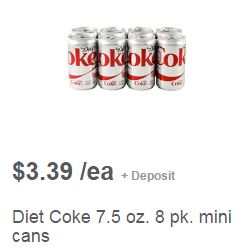This image is a cropped section from a website, displayed against a white background. It features an 8-pack of Diet Coke mini cans, each can boasting a sleek silver design with "Diet" written in black and "Coke" in bold red text. The photo is taken from a front-facing, slightly downward angle, allowing a clear view of the cans' top silver portions. Below the cans, the price "Three dollars and thirty-nine cents each, plus deposit" is prominently noted in black text. Additional details at the bottom include "Diet Coke 7.5 ounce 8 pack mini cans" also inscribed in black text.